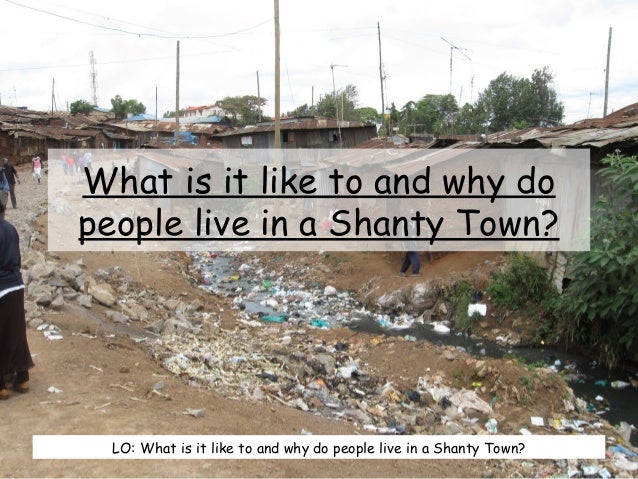The image depicts a dilapidated shantytown, characterized by a dirt path strewn with garbage, rocks, and a stream running alongside it. The scene includes makeshift structures with ramshackle roofs and wired poles for electricity, set against a sky heavy with clouds. In the foreground, people, including children, navigate up the dirt path towards the scattered houses. Superimposed on this grim backdrop, there is prominently underlined text in black Times New Roman font that asks, "What is it like to, and why do people live in a shantytown?" This primary caption is centered and displayed against a translucent white background. At the bottom of the image, a smaller white banner reiterates the question with the prefix "LO:" on the same topic. The overall ambiance reflects the dire living conditions and crowded environment of the area. The colors in the image range from various shades of brown and gray to hints of green and blue amidst the dirt, refuse, foliage, and structures.